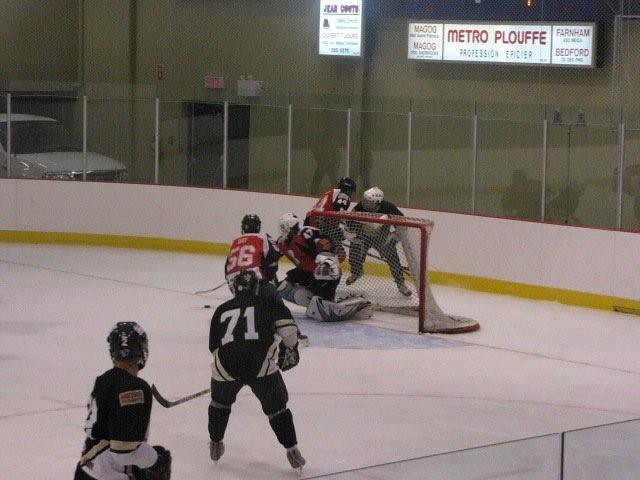This full-color indoor photograph captures an intense moment during an ice hockey game. The scene is centered around the red team's goal, where six players—three in black and white uniforms and three in red and white—are vying for control of the puck behind the net. The icy surface of the rink is prominently visible, painted underneath with the typical markings for hockey. The rink is delineated by white walls topped with glass viewing areas, with a distinctive yellow stripe running along the base of the walls.

On the far left corner of the image, part of a white truck or van is visible, parked near a door with an exit sign above it. Next to the door are two illuminated advertisement signs; the larger one reads "Metro Professional" followed by an unclear text. The overall setting, with its beige background wall and clear plexiglass partitioning, clearly indicates an indoor hockey arena. The action appears to be part of an ongoing game, as players, including what looks like a goalie, are fully engaged and the atmosphere is charged with the excitement typical of a live sporting event.